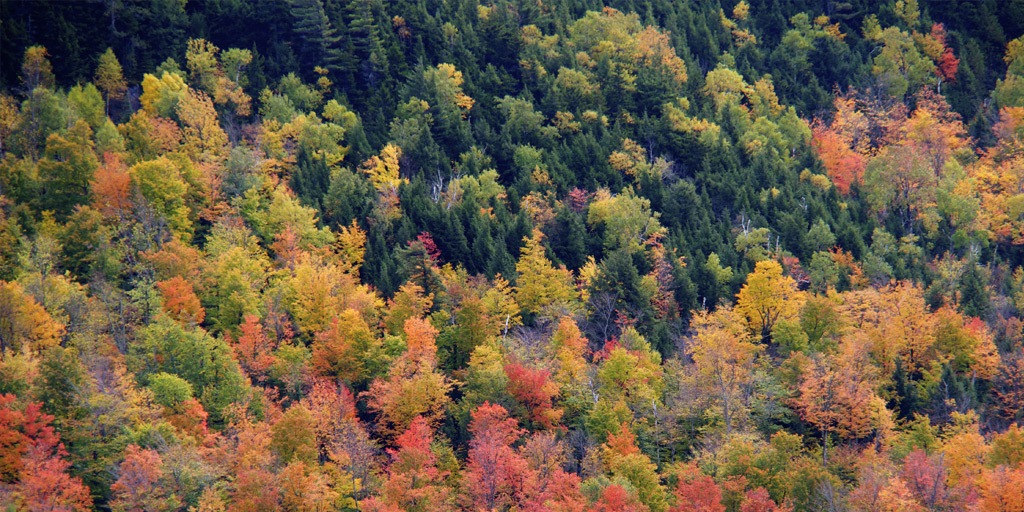This aerial photograph captures the lush and thick treetops of a forest transitioning into the fall season. The scene is vibrantly colored with a mix of greens, oranges, rust browns, salmon pinks, and darker reds dispersed among the treetops. The lower left corner of the image prominently features a dense cluster of trees that have turned vivid shades of red, yellow, and orange. As your gaze travels diagonally from the lower left to the upper right, the colorful foliage gradually fades into a strip of entirely green treetops, maintaining their summer foliage without any seasonal change. The image's upper right corner again reveals trees tinged with autumn hues. Notably, some trees appear slightly blurred, possibly due to the capture angle or movement, suggesting the photo may have been taken from a fast-moving aircraft. The upper left corner has a dark section that partially obscures the view, adding a mysterious touch to the scene. Despite the blur and the dark section, the overall image beautifully showcases the striking and varied colors of autumn foliage in a forest.